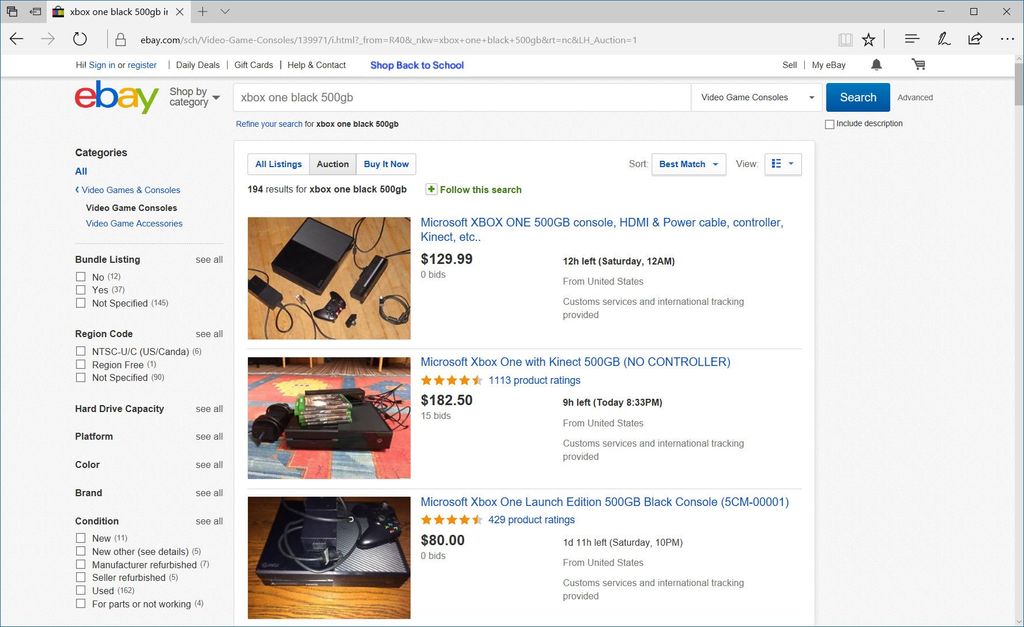This image is a screenshot taken from an eBay search for "Xbox One Black 500 GB." At the top of the screenshot, the familiar eBay logo is prominently displayed with its distinctive colors: a lowercase 'e' in red, 'b' in blue, 'a' in yellow, and 'y' in green. Below the search bar, it indicates there are 194 results for this query, although only three listings are visible in this image.

The first listing seen at the top is for a "Microsoft Xbox One 500 GB Console" which includes an HDMI cable, power cable, controller, and Kinect sensor. The listing mentions that it is currently up for bidding with 12 hours remaining, though no bids have been placed yet. The starting price is set at $129.99.

Further down, the second listing is for a "Microsoft Xbox One with Kinect 500 GB" but without a controller. This item has garnered more interest with 15 bids, driving the price up to $182.50.

Lastly, the third visible listing is for a "Microsoft Black Console" without any accessories mentioned. This listing has zero bids so far and is priced at $80. The accompanying number in parentheses is not fully visible but typically would indicate the quantity available or other relevant information.